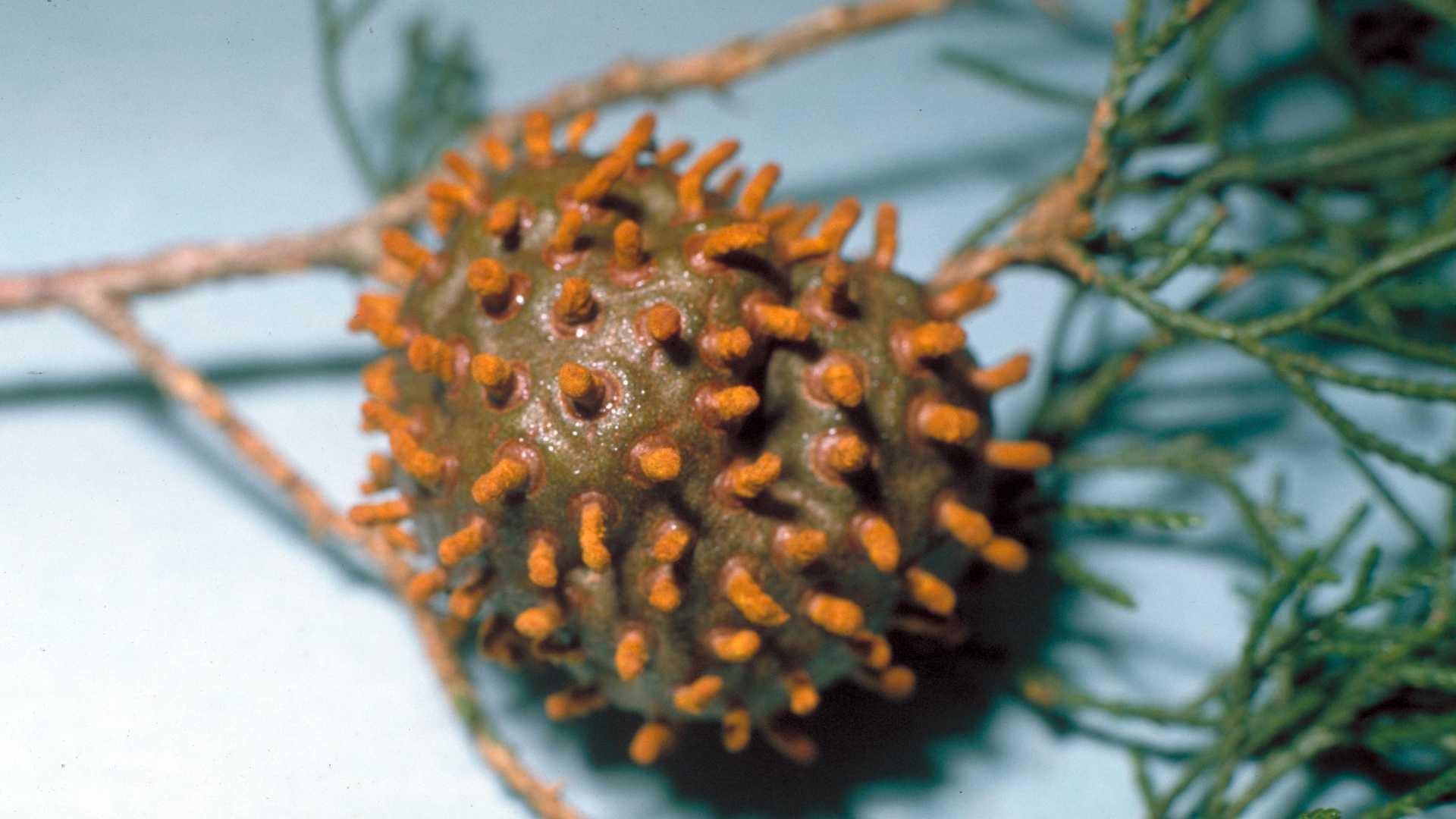The image features a close-up of a gall on a plant, resembling an irregular growth or seed pod. The gall is a brownish-green, olive-colored blob with an unsettling, almost wet or waxy appearance that reflects light, giving it an iridescent shimmer. Emerging from the gall are numerous little orange spikes, reminiscent of the texture of a coronavirus cell, adding to its bizarre and somewhat repulsive look. This growth is attached to a plant that appears to be a pine or juniper branch, identifiable by the small sprigs of evergreen leaves and branching brown twigs that are faintly visible beneath the gall. The background is a solid blue, likely a photographic work surface, adding to the object's prominence and emphasizing the detailed and unnatural appearance of the gall. In the photograph, the gall is the primary focus, while the rest of the plant and the surface it rests on are blurred, heightening the sense of its unusual and alien characteristics.